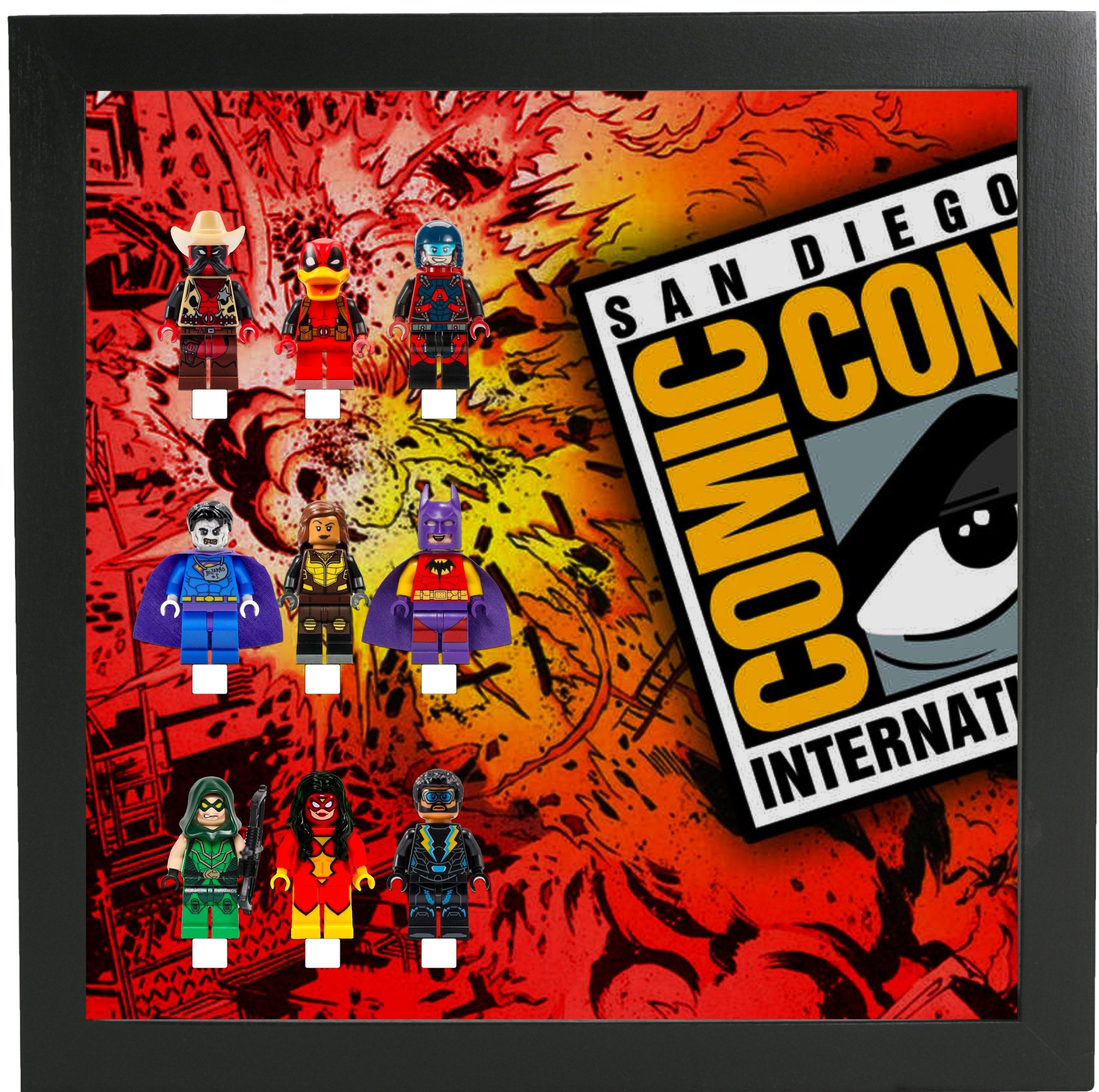The image is a detailed and vibrant comic art poster styled for cartoons, prominently featuring nine action-figure-like characters arranged primarily towards the left side, each rendered as puppets or small dolls. The background is a dynamic mix of red and yellow, depicting an explosive scene that enhances the action-packed theme. 

On the top left, there's a sheriff figure; in the middle, several figures stand out including one dressed in red and another in blue. Near the right side, a military figure is present alongside a distinctive purple Batman figure. More characters include a brown-costumed figure in the center, a green-costumed figure at the bottom left, a red and yellow figure at the bottom center, and a black figure at the bottom right. 

Additionally, the right side of the image features an inset, tilted slightly, with the text "Andy, here you go, Comic-Con International," where "Comic-Con" is prominently displayed in yellow. Near this inset is an eye with a grey face, adding a mysterious element. The overall frame of the image is dark grey, set against a white background, enhancing the comic art aesthetic.